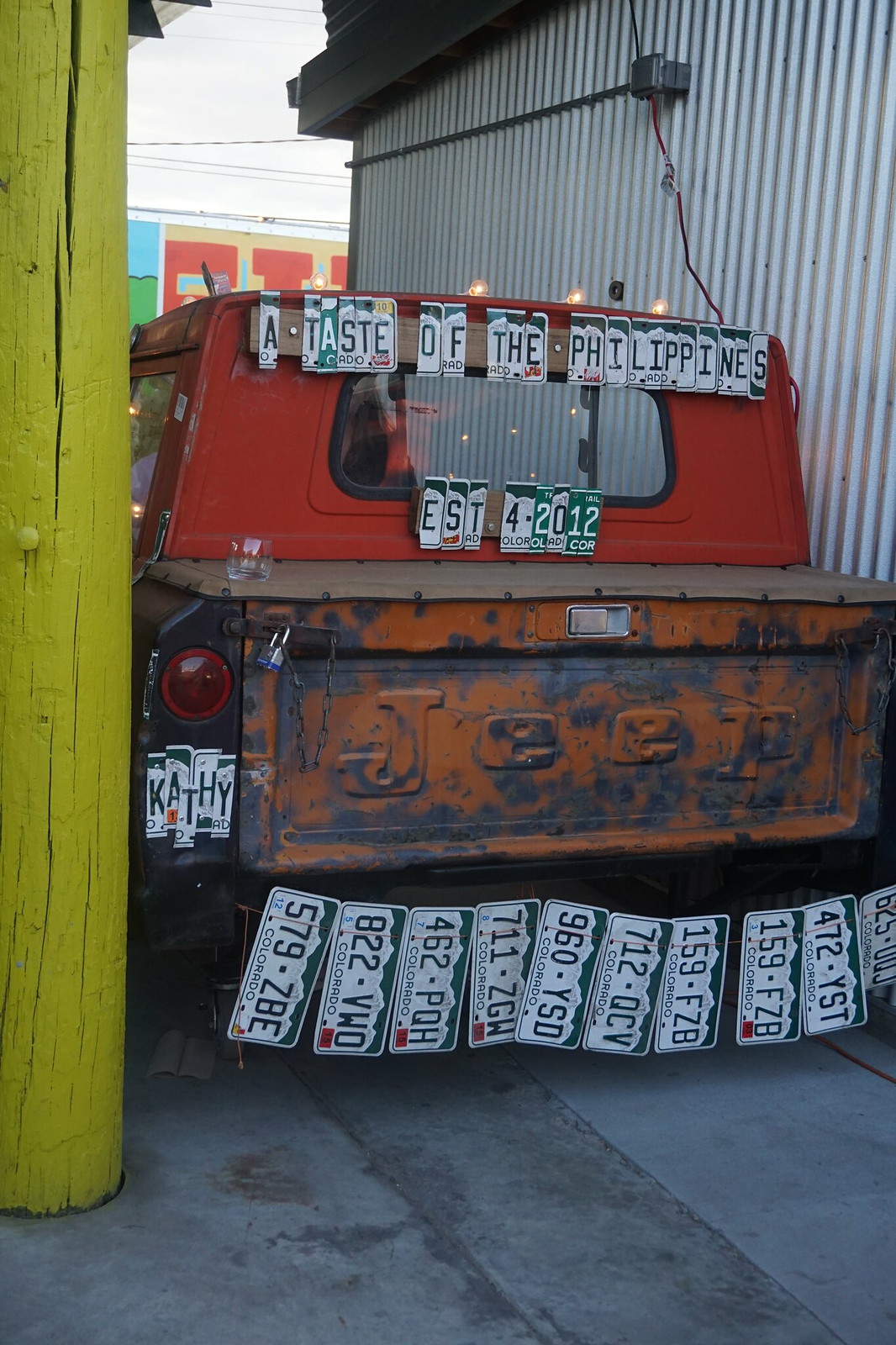The image showcases the back of a vintage, rusty Jeep pickup truck, predominantly colored in red with black and orange rust marks. The vehicle appears non-functional and serves instead as a decorative piece, given the multitude of Colorado license plates affixed to it. Centrally, the truck bears an intricate message crafted from cut-out sections of various license plates. Above the rear window, the phrase "A Taste of the Philippines" is prominently displayed, signifying perhaps a restaurant or cultural homage, with the establishment date noted as EST. 2012 just below it. Further down, the name "Cassie" or "Cathy" is similarly fashioned from license plate fragments. To the left of the truck, there’s a noticeable yellow electric pole, adding to the rustic charm and aged aesthetic of the scene.